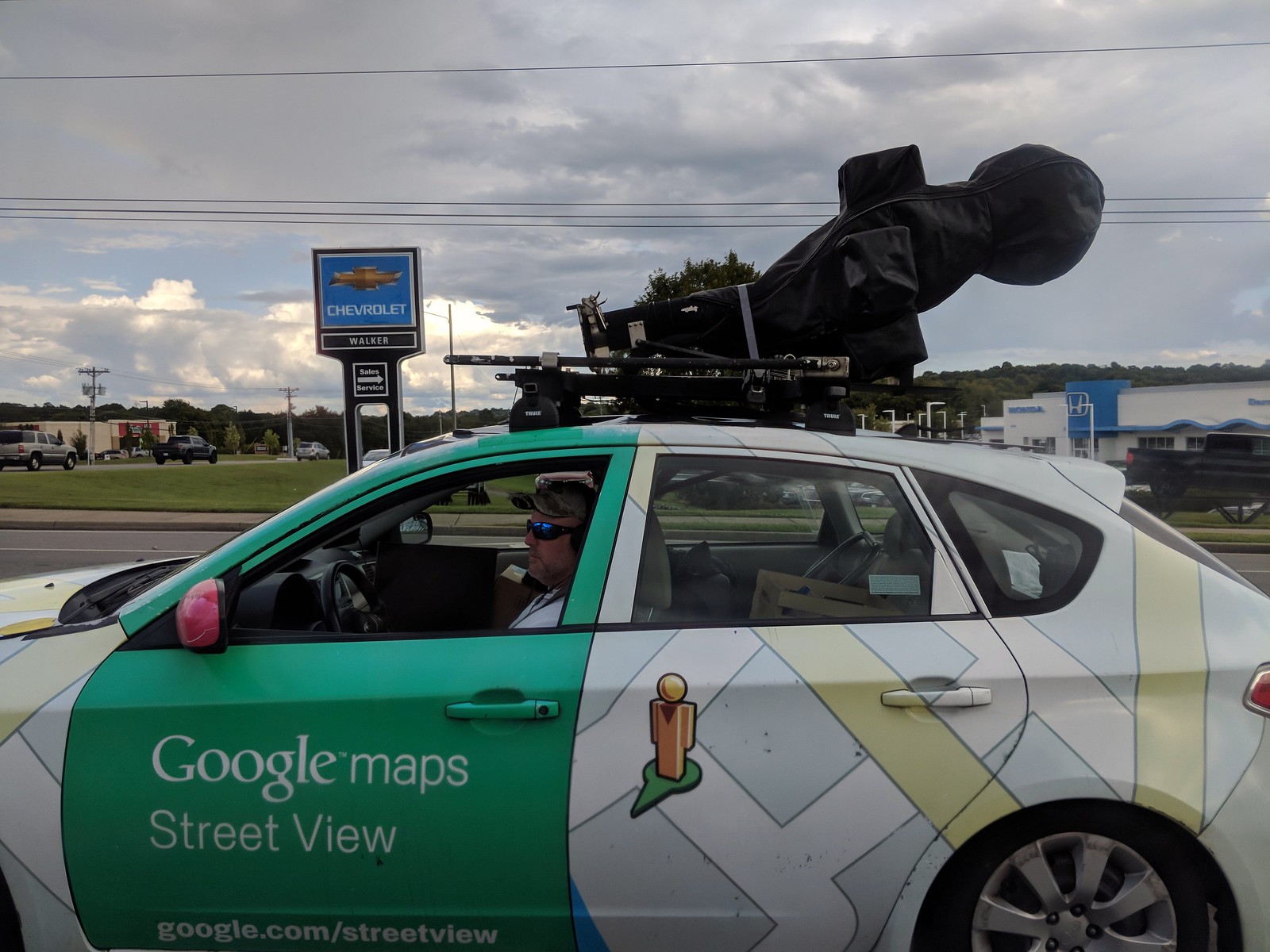The image captures an outdoor scene with a variety of details. The top portion features a sky transitioning from blue on the left to predominantly cloudy, with white clouds spreading across the expanse. In the background to the right, a building with a distinct "Honda" sign in blue lettering stands out. This white building also has a blue, round structure resembling a chimney with a silver "H" logo, indicating it's a Honda car dealership.

On the left side of the image, there's a notable billboard with a black outline and a blue center displaying the word "Chevrolet" in white, along with "Walker" written underneath. In the foreground, a car is partially visible; it is marked with "Google Maps Street View" in white lettering on the front. The driver's side of the car is green, adorned with a map-like design. Although the car is zoomed in, partial views of white and yellow lines suggest it is situated in a parking area or on a street.